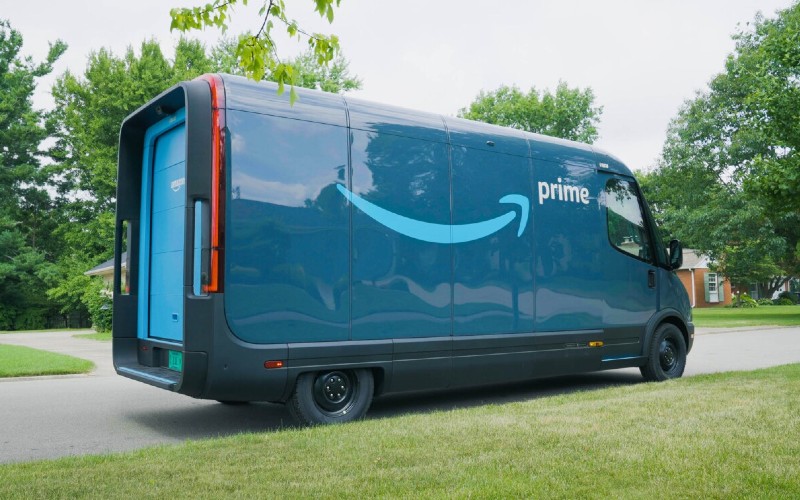This photograph captures a sizeable Amazon Prime delivery truck parked along a quiet neighborhood street. The truck, painted in a distinctive teal blue, prominently displays the Amazon Prime logo featuring a cheerful sky-blue smile and bold, lowercase white lettering. 

In the background, you can observe parts of two red-brick homes framed by large, mature trees, indicating this is an older neighborhood rich with greenery. Despite the abundance of foliage, the grass in the front yard appears somewhat dull and in need of water. 

The truck itself seems to be one of the newer models, likely equipped with air conditioning, and features a rear garage-style lifting door. Notably, a tree branch hangs low, nearly touching the top of the truck, adding a touch of natural charm to the suburban setting.